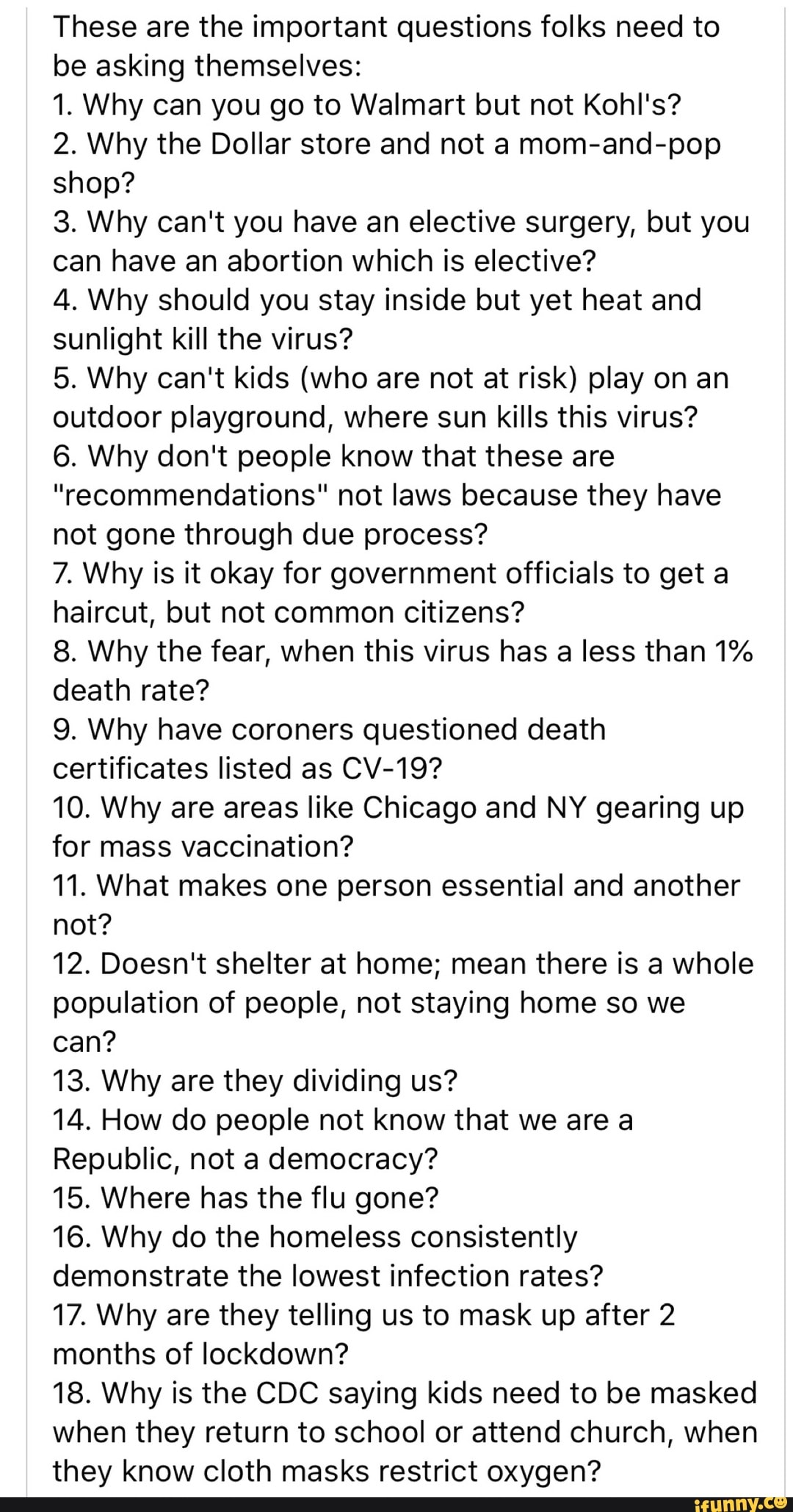The image features a cluttered white background adorned with dense black text, presenting 18 critical questions intended to provoke thought and discussion. These questions are organized in a top-right section of the image and delve into various societal and policy inconsistencies. Notable examples include: "Why can you go to Walmart but not Kohl's?" and "Why is it okay for government officials to get a haircut but not a common citizen?" The text, presented without proper spacing or formatting, makes it challenging to read. Additionally, faint vertical gray lines run up and down on both sides of the image, further contributing to the visual clutter.

The bottom of the image showcases a yellow banner with "funny.com" written in slim black text, accompanied by an exclamation mark. The overall aesthetic is chaotic, with crowded text and poor design choices that complicate readability, yet it aims to address various topics such as family, CDC guidelines, and humorous clips, though the humor may be subjective.